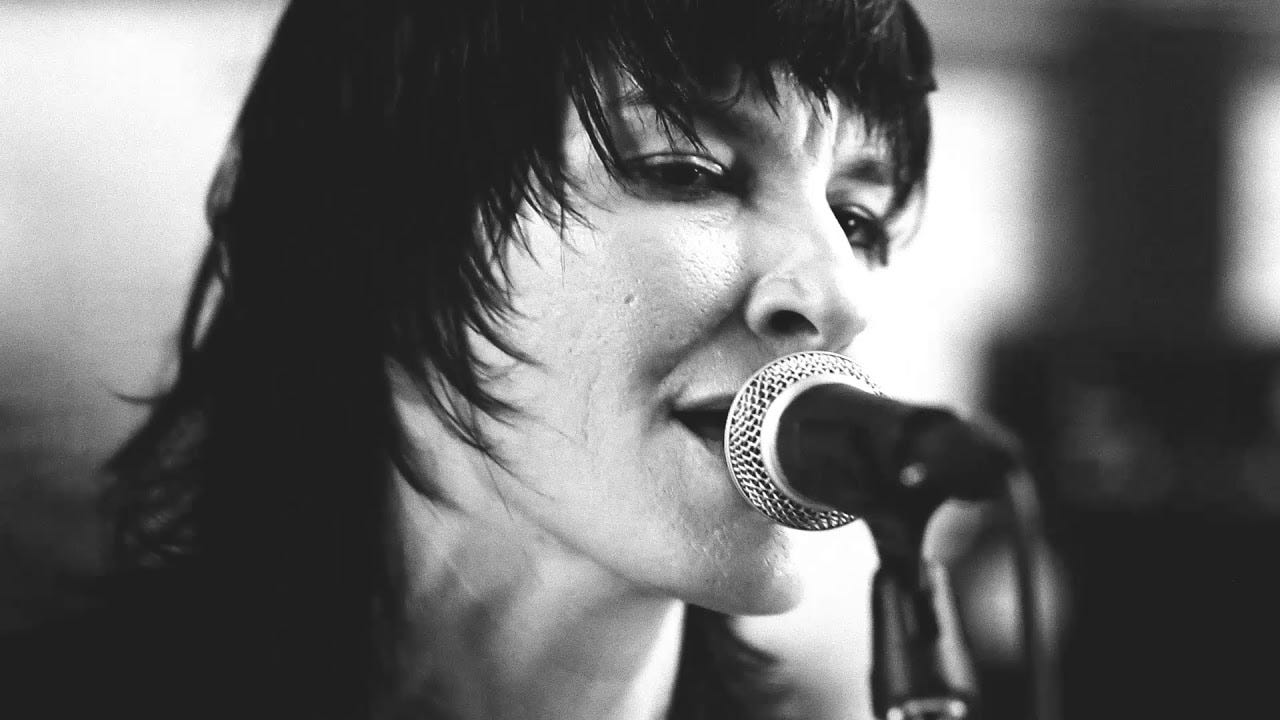In this black and white photograph, a female singer with long, dark hair down to her shoulders is captured mid-performance, singing into a black microphone with a lighter-colored tip. Her mouth is close to the microphone, nearly touching it, and she appears to be wearing red or a similar shade of lipstick. Her hair falls across her forehead, partially obscuring her face. The backdrop behind her is out of focus, dominated by contrasting shadows of black and white. The photo is cropped at her neck and chest, emphasizing her intense expression as she sings. The microphone, which features a visible silver top of its stand at the bottom right of the image, is anchored by a black electrical cord. The entire scene artfully centers on the singer's passionate engagement with her music.